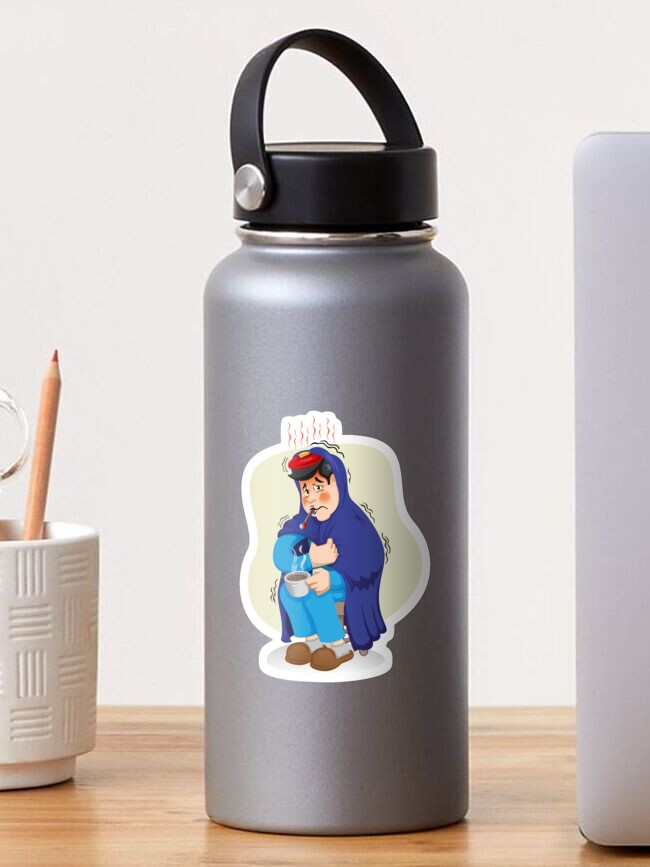This is a close-up photo of a silver metallic thermos or water bottle with a black rubber top and handle, designed to keep liquids hot or cold. Prominently featured in the center is a detailed decal depicting a cartoon character who appears to be sick. The character is bundled in a blue jacket or blanket, wearing blue pajamas, gray socks, and brown slippers, with a thermometer in his mouth and a cup of coffee in hand, looking quite miserable. The thermos sits on a brown wooden table next to a white pencil holder containing a single sharpened pencil. In the background, there's a blank white wall, and to the right edge of the image, part of a white object is visible, possibly a computer screen.